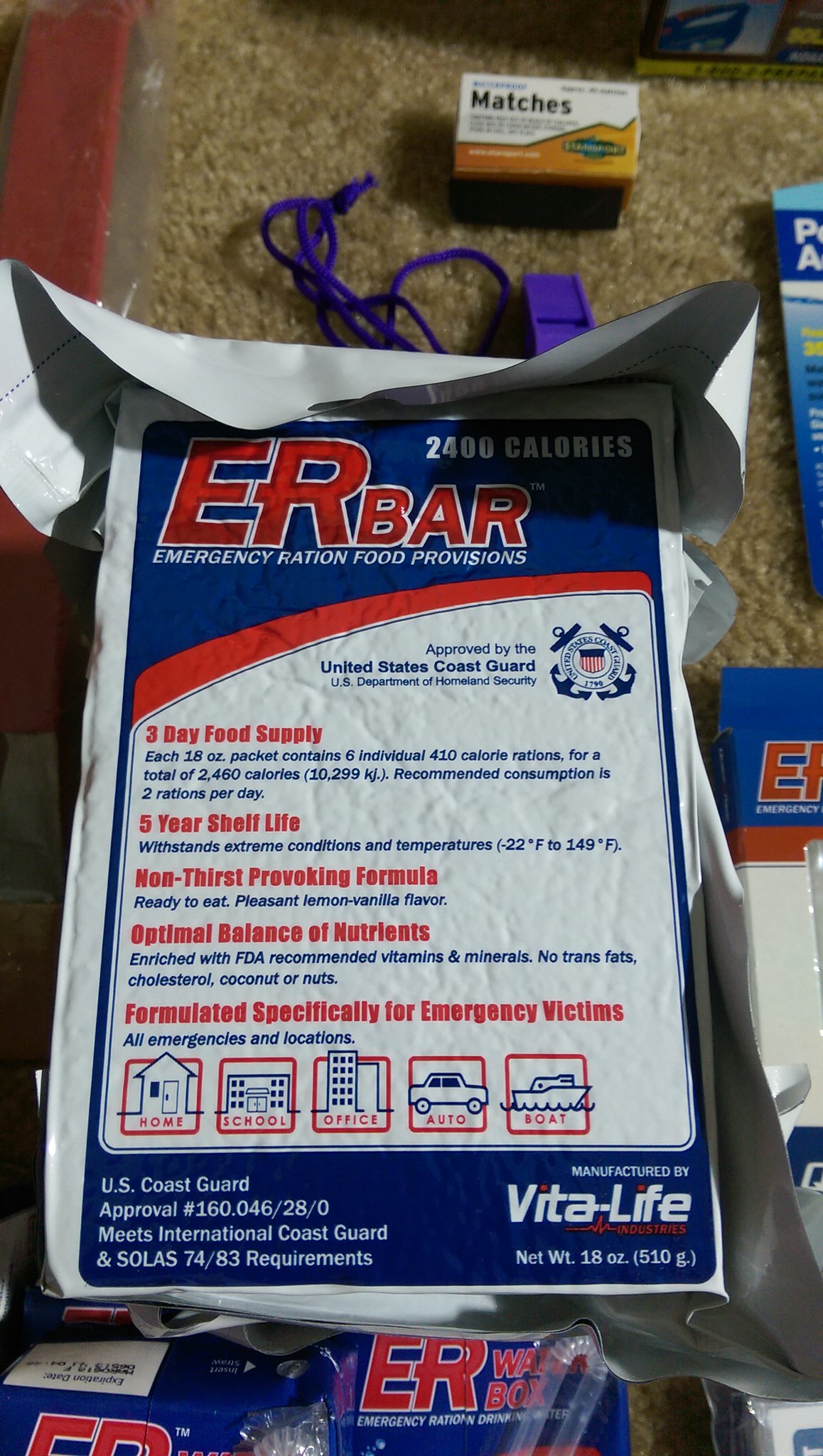The photograph is a detailed close-up of an emergency ration food provision package, prominently labeled as "ER Bar Emergency Ration Food Provisions." This vertically rectangular, unopened white package takes up about 60% of the image. It features crucial survival information in bold red and blue text, indicating it is a three-day food supply with a total of 2,400 calories, a five-year shelf life, and a non-thirst-provoking formula. The packaging claims it provides an optimal balance of nutrients, specifically designed for emergency victims, and is U.S. Coast Guard approved, meeting International Coast Guard and SOLAS 74-83 requirements. Manufactured by Vitalife, the package also highlights its features with phrases such as “optimal balance of nutrients” and "formulated specifically for emergency victims." Additional emergency items are visible around the package: a yellow and white box of matches, a purple whistle with a matching rope, and a partially visible blue package sitting on a textured brown surface that resembles carpeting. The overall color scheme of the scene includes red, white, blue, yellow, and purple elements, enhancing the visual focus on emergency preparedness.